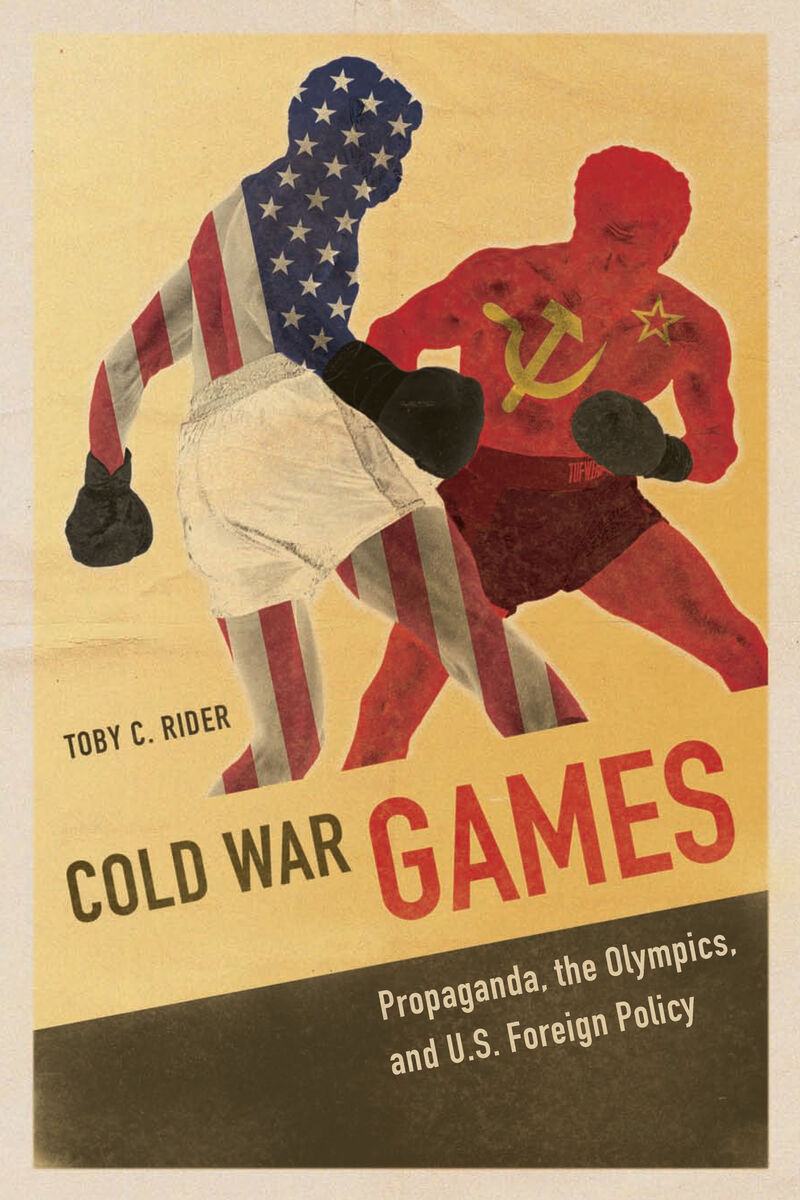The image appears to be the cover of a book or magazine titled "Cold War Games: Propaganda, the Olympics, and U.S. Foreign Policy" by Toby C. Ryder. The cover features a beige background with the bottom fifth section angled to the bottom left and colored in dark brown. In the dark brown section, the text "Propaganda, the Olympics, and U.S. Foreign Policy" is written in white. In the beige section, directly below a striking visual, the words "Cold War" are in brown, and "Games" is in red.

Dominating the center of the cover are two silhouettes of boxers in a dynamic fighting pose. The boxer on the left represents the United States, with his body covered in the American flag—white stars on a blue field over his head and shoulders, and red and white stripes extending over his torso, arms, and legs. He is wearing white boxing shorts and black boxing gloves. The boxer on the right symbolizes the Soviet Union, depicted entirely in red with distinct Soviet symbols: a yellow hammer and sickle and a star on his left shoulder. This Soviet boxer is crouched low, seemingly ready to take a swing, facing slightly sideways and away from the viewer. Together, these elements convey a striking representation of Cold War tensions and ideological conflict.